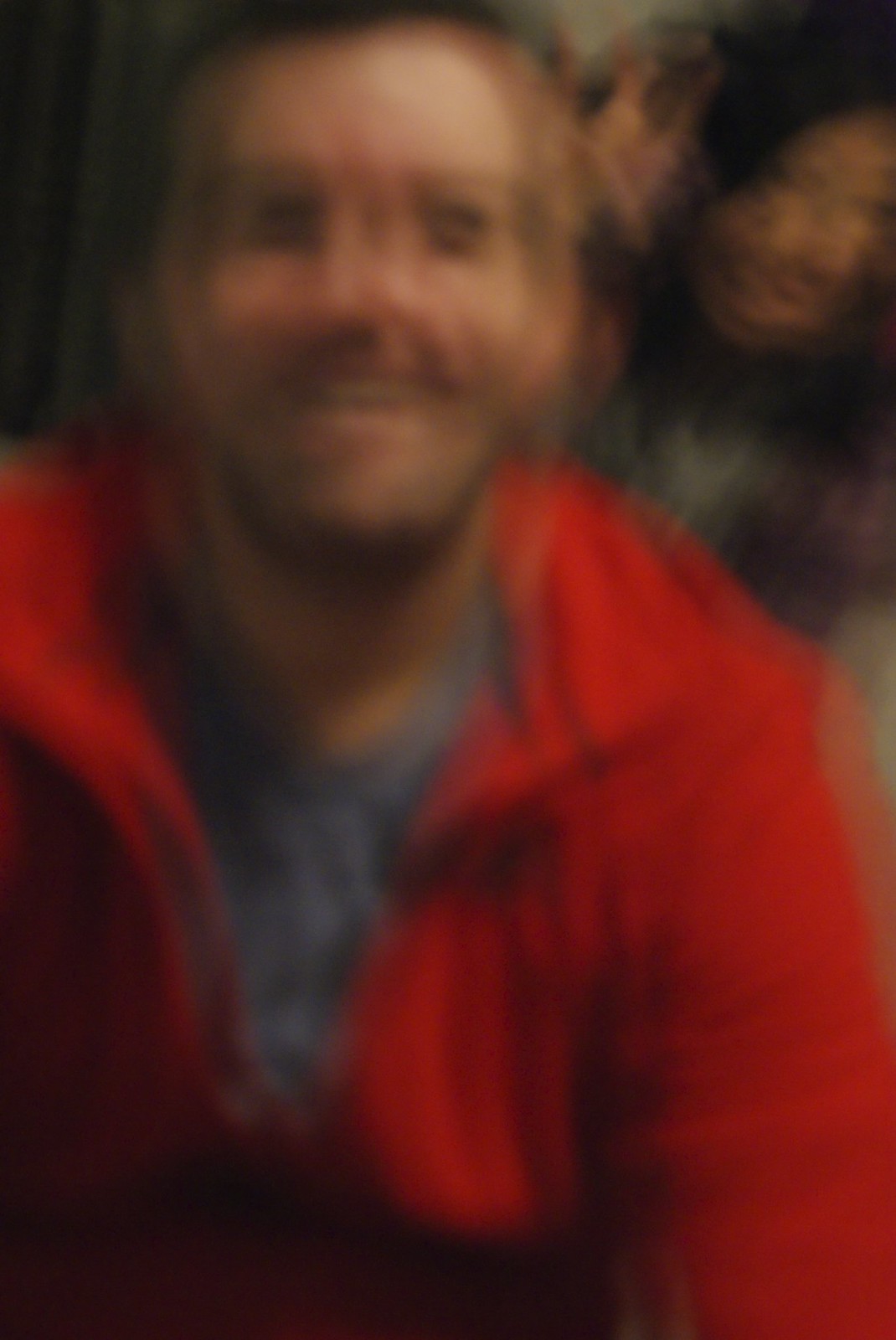A vertically oriented photo captures a moment shared between two individuals, although the picture is unfortunately plagued by significant blurriness that suggests either a camera malfunction or subject movement. The background is indistinct, making it challenging to determine whether the scene is indoors or outdoors, especially given the lack of a defined light source. The upper left corner of the image appears especially dark.

The focal point of the picture involves two people. Despite the blurriness, the outline of a woman with dark hair is discernible; she appears to be gesturing with a peace sign behind a man, adding a playful element to the scene. The man, outfitted in a red jacket over what seems to be a gray shirt, has reddish auburn hair, a beard, and a goatee, and he is smiling directedly at the camera. The woman’s ethnic origin is ambiguous, though she might be of Asian descent. The overall image conveys a spirited interaction between the two subjects despite the unclear setting and blurred details.